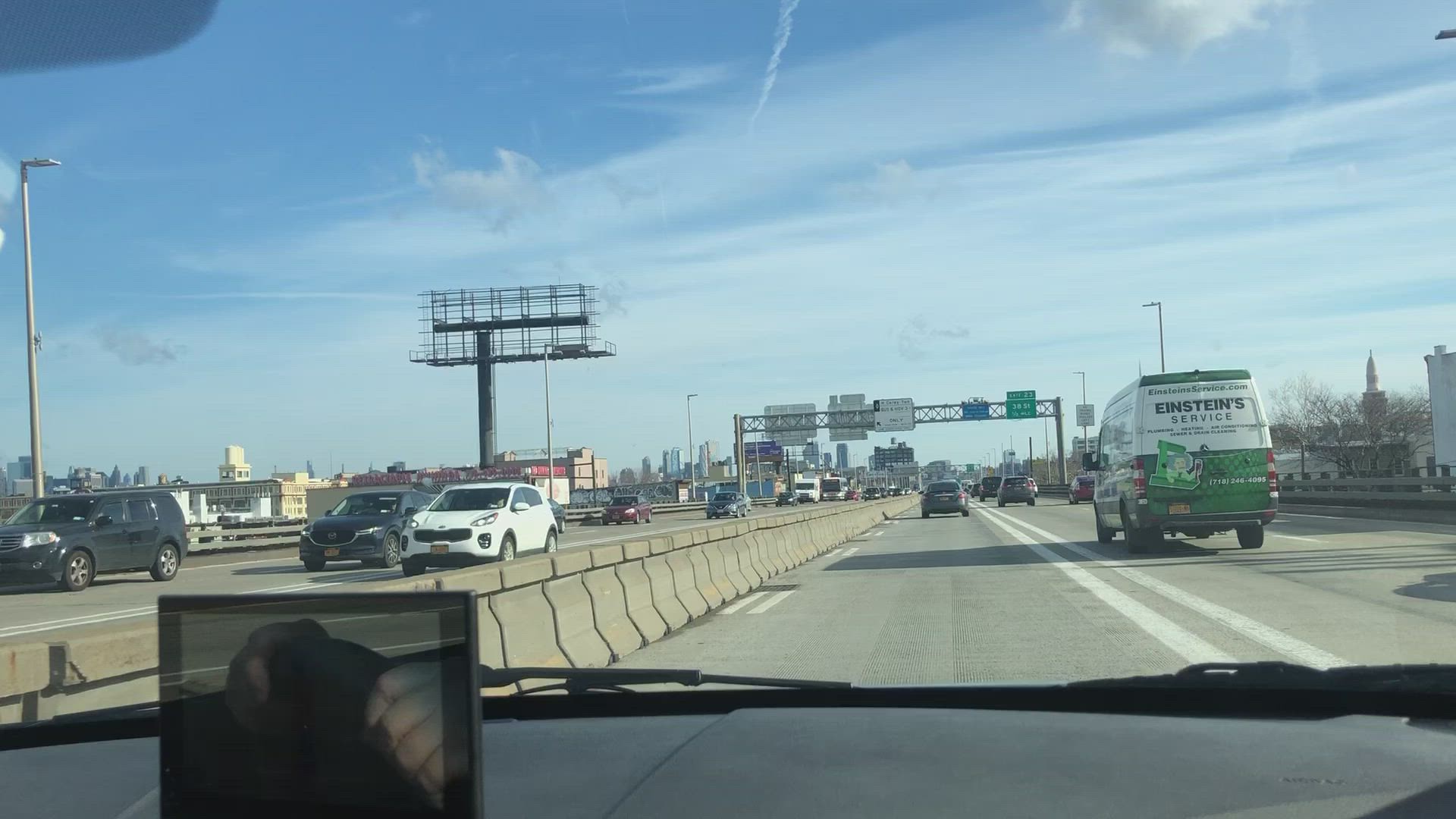This photograph, likely captured from a dashcam or mobile phone camera, depicts a bustling six-lane highway, with three lanes in each direction separated by a concrete median barrier. The road is populated with various vehicles in hues of dark gray, dark blue, and white. Notably, a green and white company van is driving in the right lane. The sky above is a mix of clear blue and scattered clouds, suggesting a partially overcast day. Visible on the sides of the image are parts of the car's interior, possibly including a reflection of the driver in a small panel on the left. The driver's hand is seen gripping the steering wheel on the right side of this panel, further emphasizing the in-action capture of the scene.